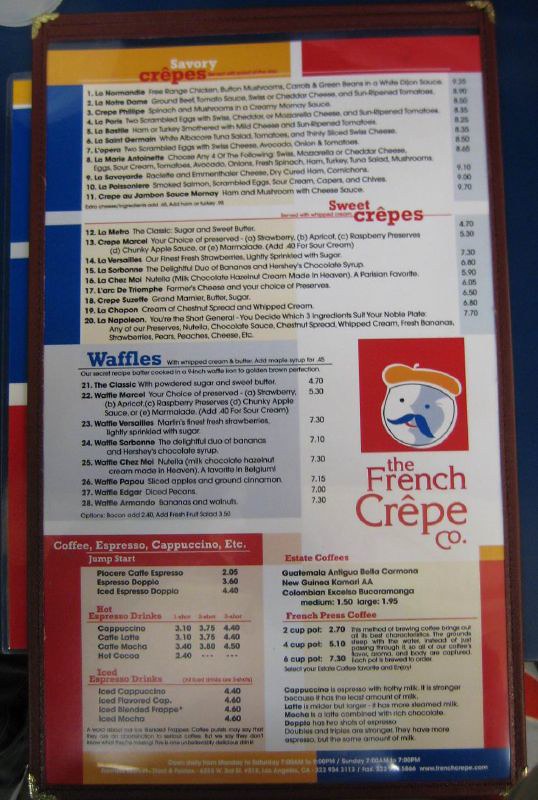The image showcases a detailed menu from "The French Crepe Company, CO." The menu is elegantly divided into various sections, focusing primarily on their signature offerings. At the top portion of the menu, there's a delightful array of crepes, segmented into savory and sweet choices. Each category boasts a variety of options to cater to diverse palates. Below the crepes, a section dedicated to waffles presents multiple tasty variations.

On the bottom left of the menu, there's a comprehensive list of beverages, highlighting different types of coffee, including espresso and cappuccino. The bottom right also features additional coffee selections, ensuring there's something for every coffee aficionado.

The menu's color scheme exudes a French aesthetic with hues of orange, red, and blue. The restaurant's logo is prominently displayed, depicting a whimsical face adorned with a blue mustache and an orange-yellowish painter’s hat, adding a playful charm to the overall design. The menu itself is set against a blue table background, enhancing its visual appeal.